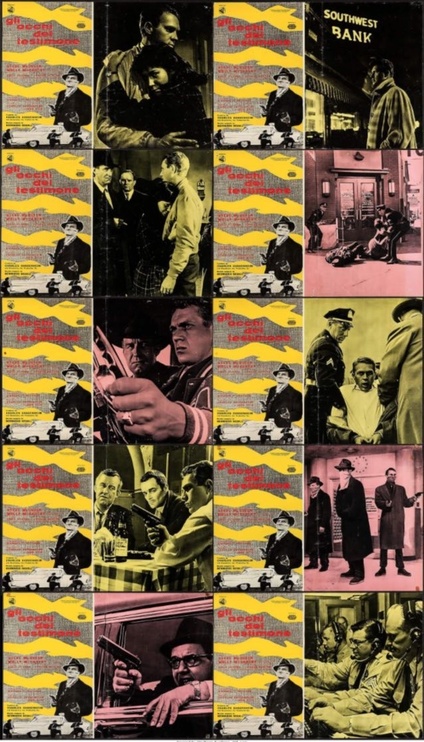The image is a meticulously arranged collage featuring a grid of 20 black-and-white photos, reminiscent of a vintage film montage. The grid is composed of five rows, each containing four images. A recurring photograph appears ten times: this picture shows a man in a black hat wielding two guns, with a white car partially shielding three men in the background. The caption on this repetitive image reads, "Gli occhi dei miei," which appears to be in a foreign language.

Other images in the collage include various action-packed and dramatic moments, likely extracted from a classic movie. These additional scenes depict:

1. Several men gathered around a table.
2. A man firing a gun through a car window.
3. A man standing in front of a building labeled "Southwest Bank."
4. A tender moment where a man and a woman are embracing.

Each photograph captures different characters in distinctive poses, encapsulating the essence and style of an old-fashioned cinematic narrative.